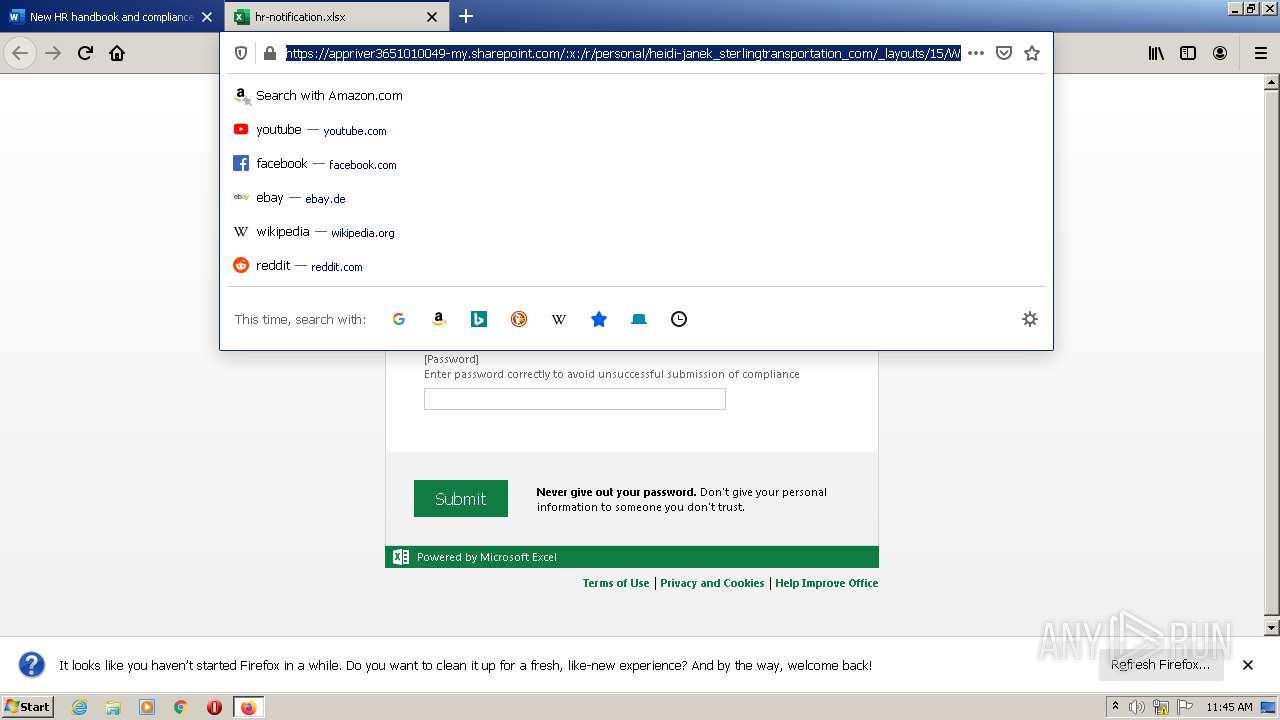A classic Windows computer screen with an active web browser, likely Internet Explorer, evocative of the late 1990s era, predominantly Windows 98 or Windows 95. The browser window is framed with vintage UI elements, a hallmark of these early Windows operating systems. There are two open tabs, a feature not as ancient, suggesting a more contemporary browser designed to emulate the retro aesthetic, possibly an older version of Firefox or even a modern browser configured to appear nostalgic. The current web address appears to be SharePoint, though it’s slightly unclear due to the small font size. The address bar is highlighted, ready for a new input, accompanied by modern search suggestions such as YouTube, Facebook, eBay, Wikipedia, and Reddit. The backdrop is a light gray, typical of the era’s design, and the user seems poised to enter a new URL.